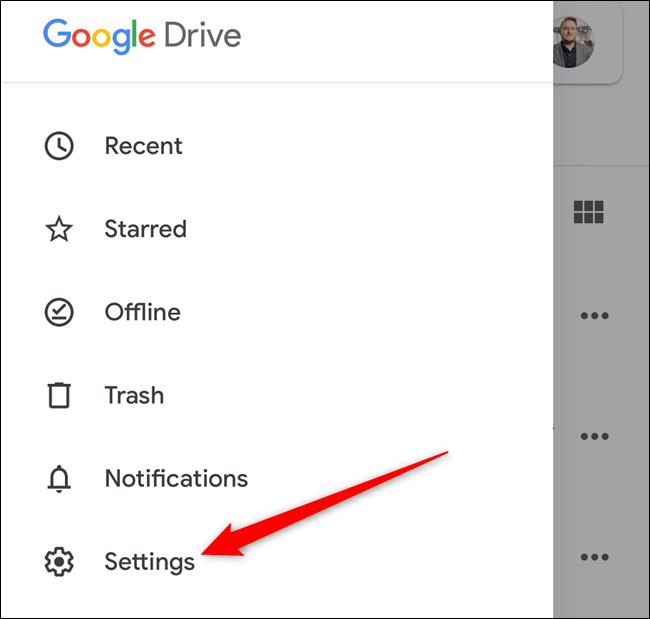A screenshot of a Google Drive interface is displayed as part of a tutorial. The image highlights the main navigation pane with tabs labeled "Recent," "Starred," "Offline," "Trash," and "Notifications." A prominent red arrow points to the "Settings" option, indicating a specific area of interest. The Google Drive logo with its colorful lettering is visible in the top section of the screen. To the right, a portion of the screen is dimmed or grayed out, suggesting an area not in focus for this tutorial. Additionally, a user's avatar is seen at the top-right corner. This detailed visual guide appears to be part of an instructional response, aiming to assist users in navigating to the settings within Google Drive.